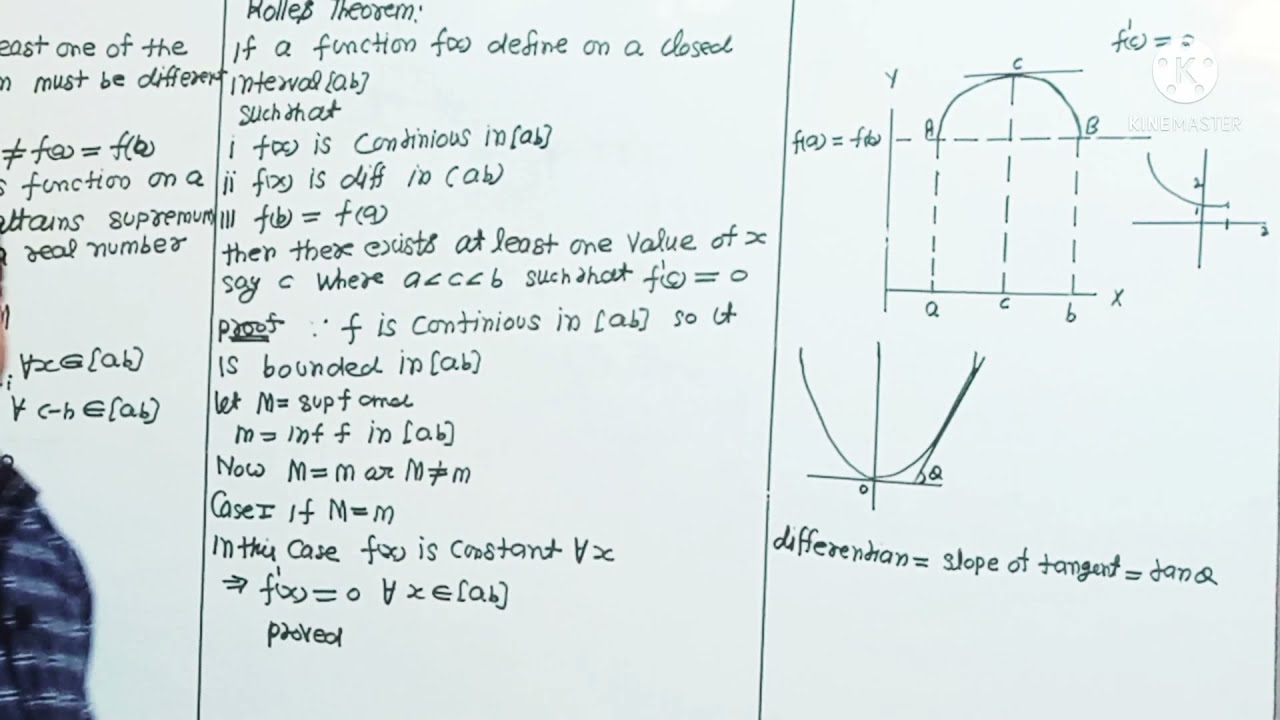The image features a whiteboard divided into three distinct sections, all written in green ink. The leftmost section contains a mix of words and mathematical equations, with more emphasis on text at the top and equations at the bottom. The central section is filled with definitions and explanations, prominently displaying the phrase, "if a function to define on a closed interval," although some of the writing beneath this is not fully legible. The rightmost section showcases a graph with a labeled X and Y axis, indicating points C, B, and A, and includes dotted lines and various mathematical equations, such as "differentiation equals slope of tangent." There are also complex equations like F(A) = F(...) scattered around this section. Additionally, the image captures a partially visible person on the left side, identifiable by their blue striped jacket and left shoulder. The overall scene presents a detailed mathematical discussion or lecture, with numerous symbols, graphs, and textual explanations spread across the whiteboard.